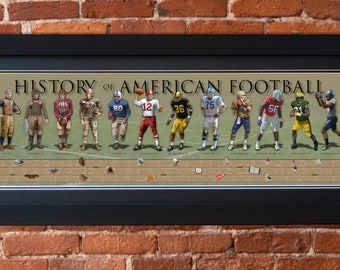A poster is tacked up on a red brick wall, displaying the evolution of American football uniforms through history. The poster, framed in black at the top and bottom, prominently reads "History of American Football" at the very top. It functions as a timeline, showing 12 different football uniforms worn from the earliest days of the sport on the left to the most modern on the right. Each uniform is worn by illustrated football players, complete with numbers on their chests. Beneath each figure, key dates and information are listed, providing a detailed progression from as early as the 1900s through to the 1980s, 1990s, and modern day. The poster's colors are predominantly red, black, and the varied hues of the uniforms themselves.